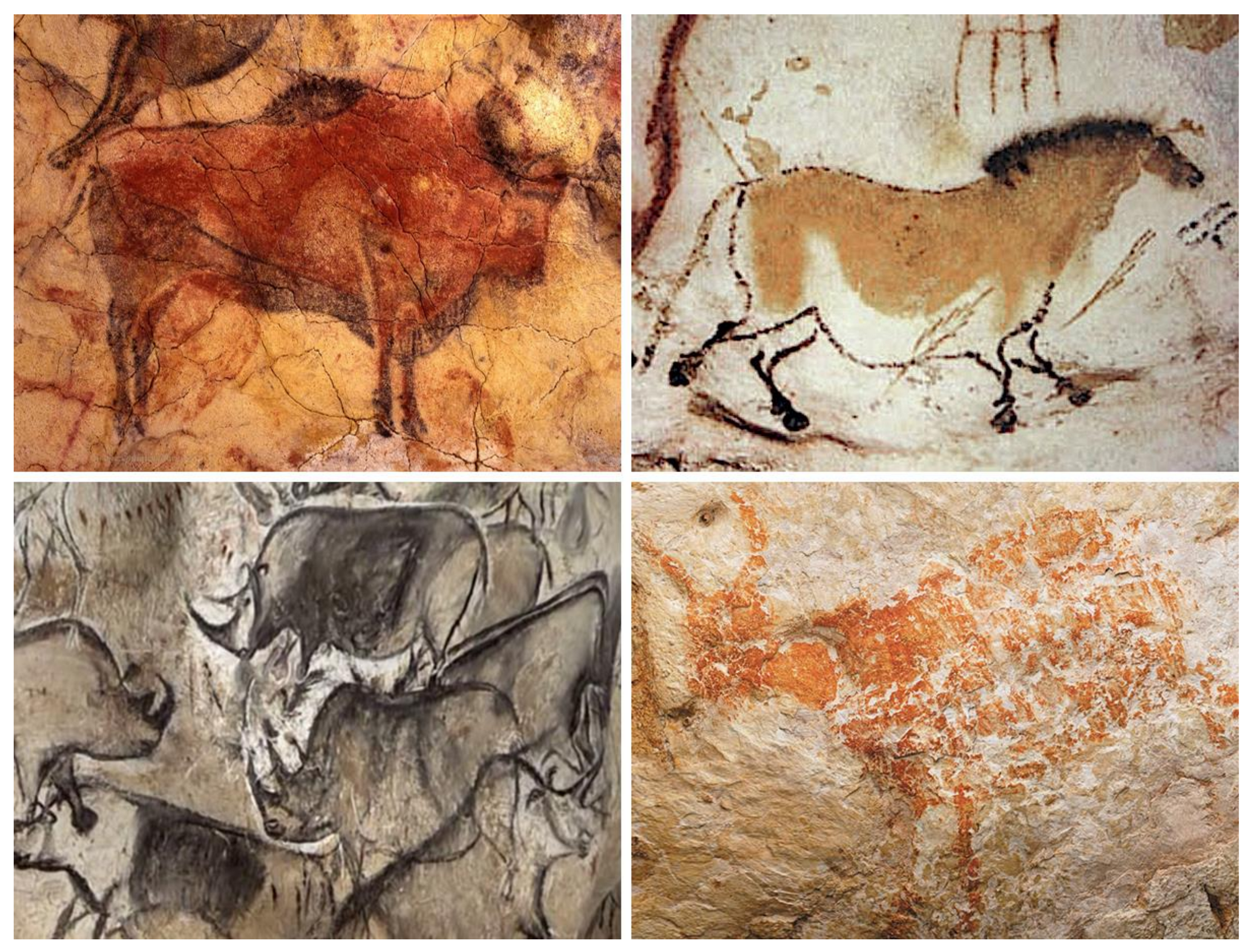This image showcases four evenly spaced photographs of ancient cave art, symmetrically arranged in a grid-like pattern. Each photograph depicts various animals rendered in distinctive styles on different colored rock surfaces. 

The top left photograph features a highly weathered, dark yellow rock wall adorned with a reddish-brown drawing of what appears to be an ox, water buffalo, or bull, facing to the right. 

To the right of this, the top right photograph presents a large brown horse, seemingly in motion, with a black mane. The horse is drawn on a white, worn wall with a possible representation of an arrow emerging from its rump, rendered with brown and white detailing. 

The bottom right photograph displays several rhinoceroses on a white rock surface, distinguished by their brown coloration. Among them, one is facing to the right while the others face left, contributing to a sense of dynamic composition. 

The bottom left photograph depicts a more abstract drawing of an antelope or similar horned animal in black and ochre pigment on a prominent white rock surface. This collection of images captures a rich variety of prehistoric art, offering a glimpse into ancient visual expressions and their naturalistic subjects.